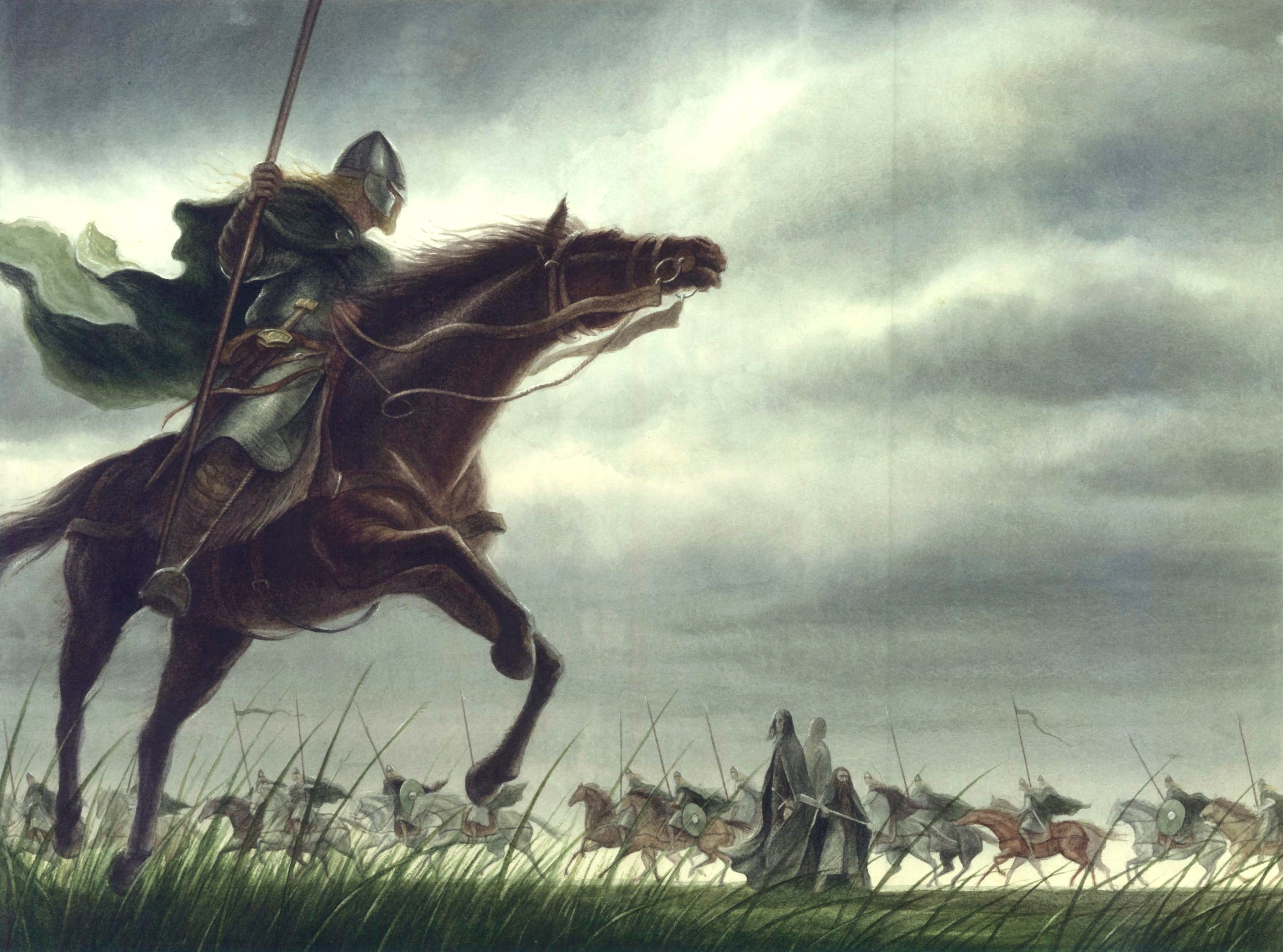A dramatic and dynamic scene unfolds under a vast, cloudy sky that dominates the upper portion of the image, stretching almost to the bottom. The foreground features a field of both shorter and longer grass, creating a rich tapestry of greens. In the background, a procession of figures and horses moves across the landscape. 

Several horses of varying colors—gray, brown, reddish-brown, and white—carry riders. Among the riders, some hold shields, while others carry distinct banners or lances, adding a sense of historical or martial significance to the scene.

In the forefront on the left-hand side stands a large, imposing brown horse, much larger than the others. A man atop the horse captures immediate attention. He is adorned in a green cape, with a shield on his head, and wields a lance or spear in his hand, though the top of the weapon is out of the frame. His outfit comprises green pants and long brown boots, enhancing his authoritative presence.

Anchoring the composition, this central figure and his mount dominate the visual space, their hooves firmly planted in the grass, grounding the scene in a vivid and immersive depiction of a historic or ceremonial moment.